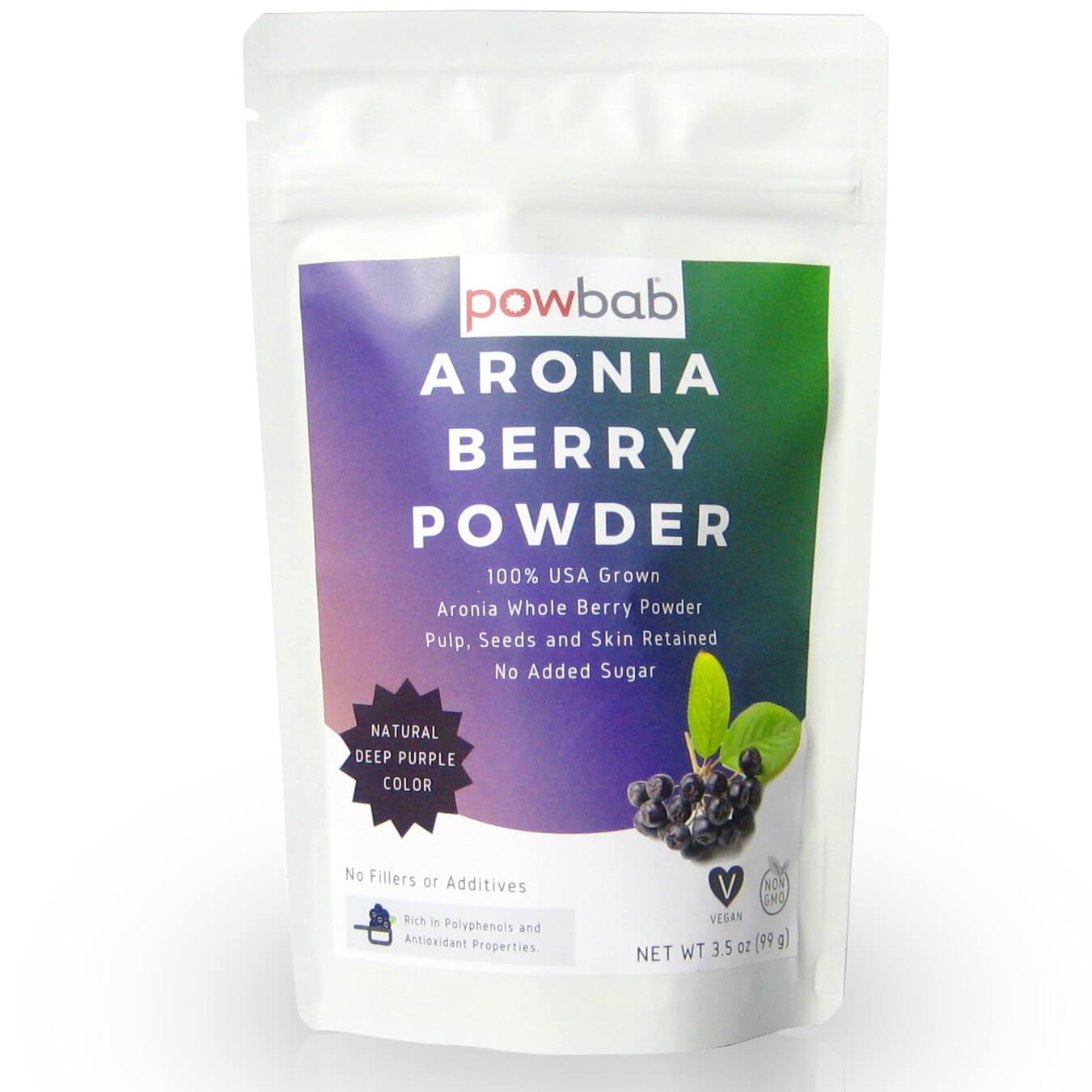The image showcases a white, sealed resealable pouch package of a product against a plain white background. The pouch measures approximately five inches in height with a width that increases from three inches at the base to four inches at the top. A notable feature is a notch on the left side, indicating a tear-open mechanism, and a raised area below it for resealing.

The design on the pouch's front includes a rectangular gradient that starts with light purple in the lower left corner, transitioning through darker purple and blue, and ending with green in the upper right corner. At the top of this gradient, a white rectangle features the brand name "POWBAB" with "POW" in red or orange letters and "BAB" in gray. Below this, in large white print, is the product name "Aronia Berry Powder."

Additional text in smaller white letters reads "100% USA grown Aronia Whole Berry Powder," followed by the statement "Pulp seeds and skin retained; no added sugar." To the left of these details, there's a black starburst with white text proclaiming "Natural Deep Purple Color." Further down on the left side, the pouch states, "No fillers or additives, rich in polyphenols and antioxidant properties." On the right side, there's an image of the Aronia berries, which are blackish in color and accompanied by two green leaves. Additionally, the lower right corner includes logos indicating the product is vegan and non-GMO, alongside the net weight information: "3.5 ounces (99 grams)."